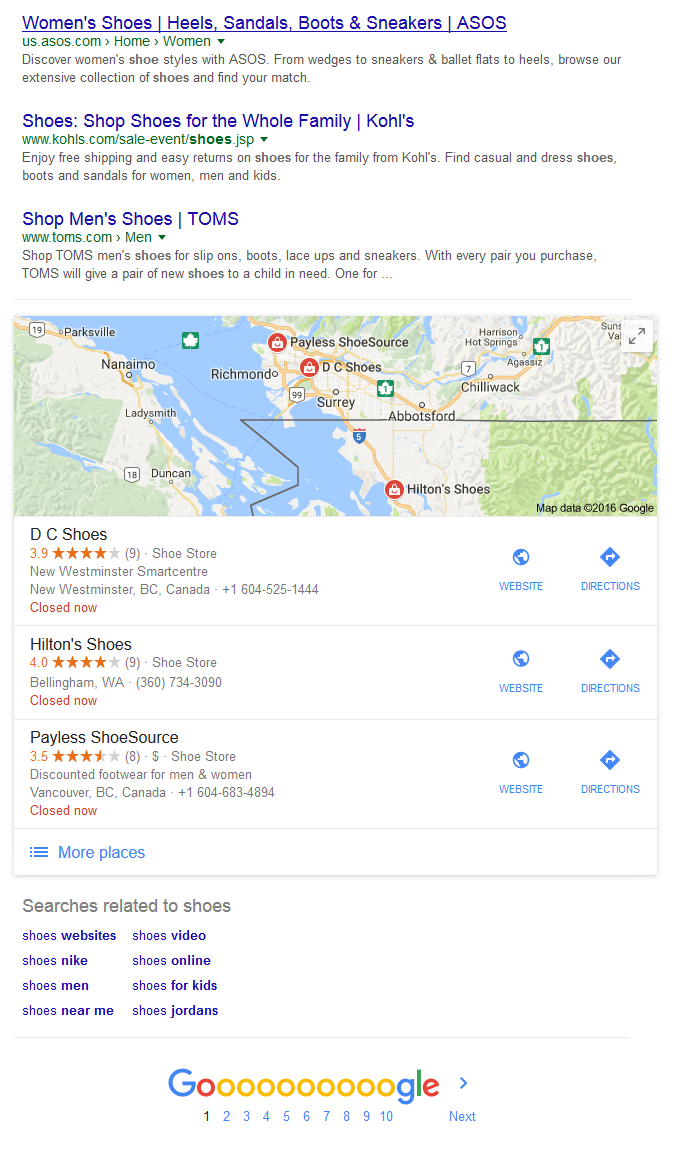This screenshot captures an informative webpage highlighting various women's shoe styles available at ASIS. At the top, a blue hyperlink reads, "Women's Shoes, Heels, Sandals, Boots, and Sneakers. ASIS. US.ASIS.com." The accompanying text invites visitors to "Discover women's shoe styles with ASIS, ranging from wedges to sneakers and ballet flats to heels. Browse our extensive collection of shoes and find your perfect match."

Central to the image is a street map displayed in light blue, light green, and beige tones. Prominently featured are the cities of Richmond and New Westminster in British Columbia, Canada. The map pinpoints several shoe stores, including Payless Shoe Stores and DC Shoes. 

Highlighted below the map, DC Shoes' listing shows a rating of 3.9 stars based on 9 reviews and is located within the New Westminster Smart Centre. The store is currently noted as closed. Further down, Hilton Shoes is displayed with a higher rating of 4 stars from 9 reviews, also indicating a store in the same region.